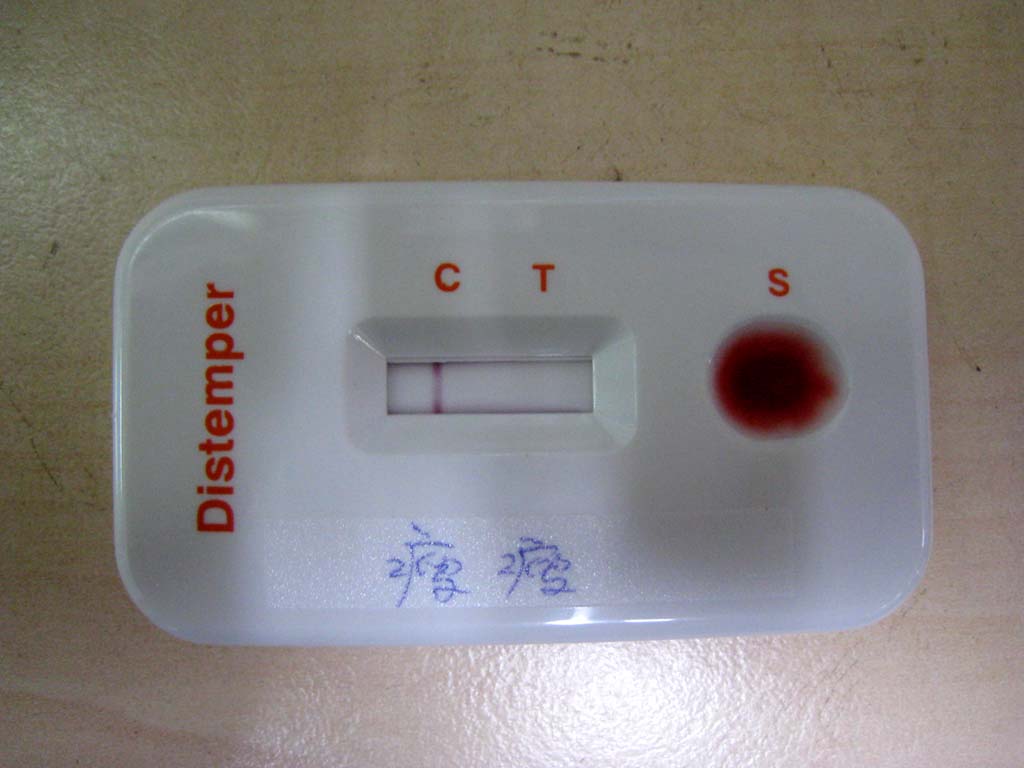Indoor close-up photograph of a medical diagnostic test for distemper on a tan countertop. The central white plastic device features rounded edges and contains a rectangular viewing window. Inside the window, there's a single vertical purple line on the left side against a white background. Above the window are two capital letters: 'C' on the left and 'T' on the right.

To the left of the viewing window, the word "Distemper" is printed diagonally. On the right, there's an oval symbol resembling a drop of blood, directly above the letter 'S'. Handwritten in blue pen on the lower half of the device are arithmetic division equations, though the specific details are indistinct.

The background and foreground are clean, with no additional text or print visible, and appear slightly illuminated by the surrounding light. The photograph seems to capture a diagnostic test, with 'C' likely indicating the control line and 'T' possibly signifying the test line, while 'S' might denote the sample area.